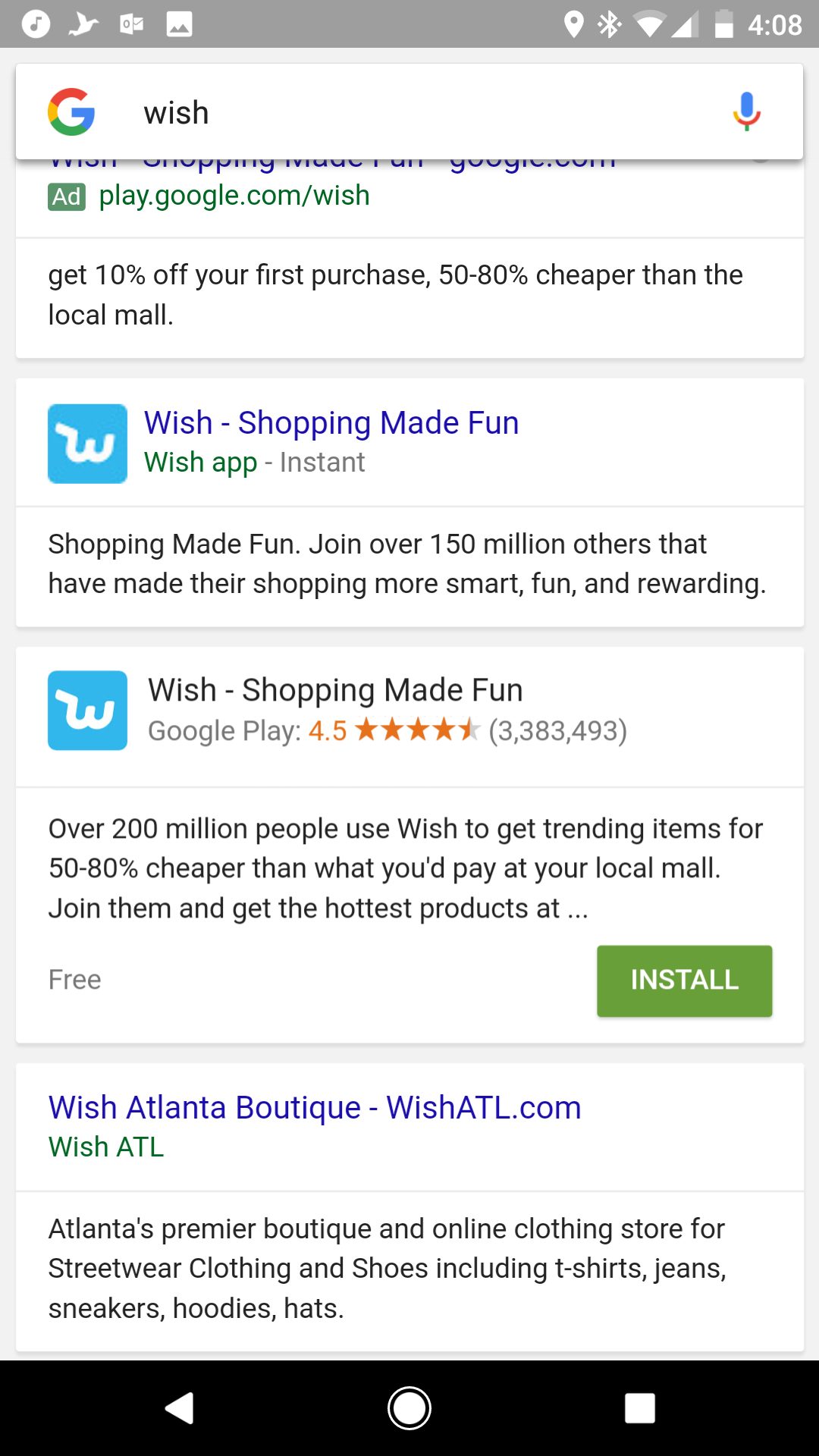This is a detailed caption for the image you described:

"A cell phone screenshot displaying a Google search for 'Wish' in the search bar at the top of the screen, just below the standard cell phone icons for battery, signal, and notifications. The screenshot reveals four search results. The very top result, partially obscured by the search bar, is an ad for play.google.com/wish offering 'Get 10% off your first purchase.' Following that, the second result is titled 'Wish - Shopping Made Fun' and references the Wish app. The third result is similarly titled 'Wish - Shopping Made Fun' and includes a green 'Install' button at the bottom of the snippet, indicating it is an app listing. The fourth and final result is for 'Wish Atlanta Boutique.'"